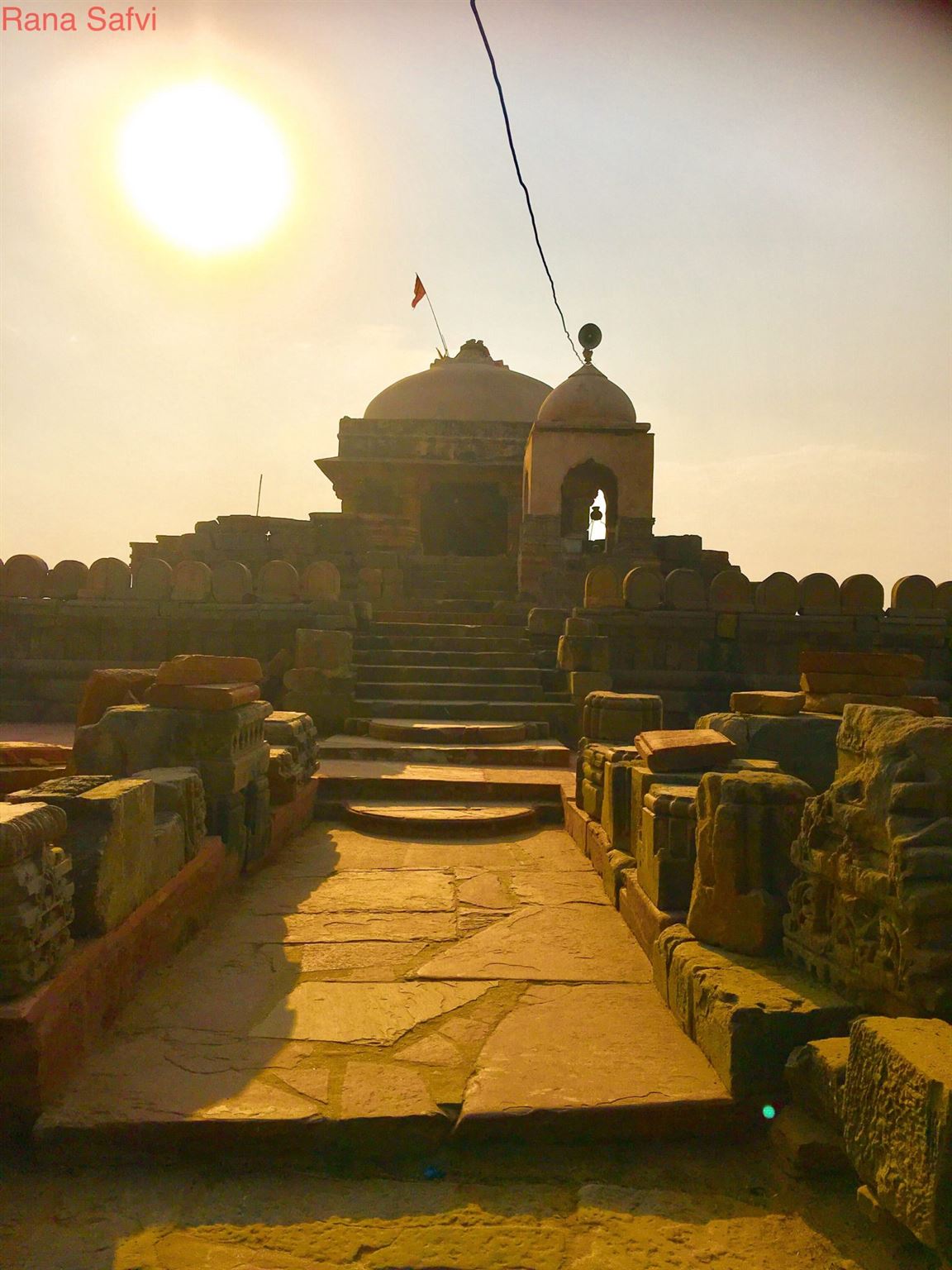This photograph captures an outdoor setting bathed in the muted brown and sandy hues typical of Middle Eastern architecture, accented by a glowing golden and blue sky at sunset. Dominating the scene are two small domed stone structures along the horizon, the larger of which, on the left, proudly flies a red flag. The smaller structure on the right features a cord or wire extending upwards. Central to the image is a wide stone pathway bordered by uneven stone bricks, guiding viewers up a series of stone steps towards the domed buildings. The meticulous stonework, consisting of various sun-baked bricks and limestone, showcases intricate, albeit indistinct, designs around the domes. Positioned in the upper left corner, red font spells out "Rana Safi," further emphasizing the Middle Eastern essence of the setting. Illuminating the entire composition, the sun shines brightly from the top left, casting a serene yet vibrant light over the scene.